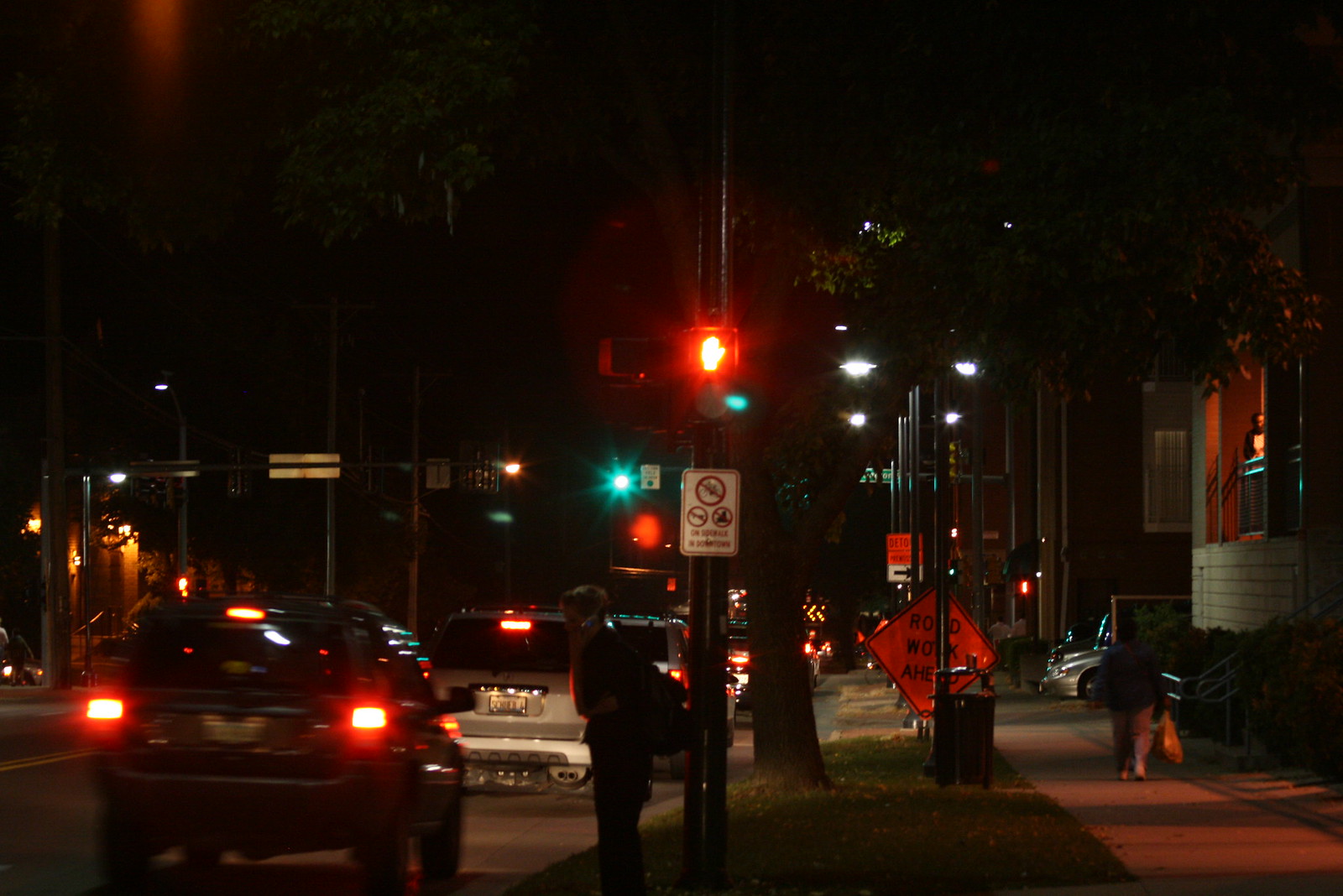This nighttime street scene captures a bustling urban atmosphere. In the bottom right-hand corner, a sidewalk stretches alongside illuminated buildings, casting a warm glow. A diamond-shaped orange sign reading "Road Work Ahead" is partially obscured behind a light pole on the left side of the sidewalk. Further down the street, additional light poles illuminate the path, along with an unreadable street sign.

Visible on the left side of the image is a person walking towards the viewer, carrying a bag. The low light obscures their face, adding an air of mystery. Centered in the middle of the scene, another individual stands next to the curb under a "Walk" sign, marking a crosswalk. Traffic fills the street, with cars moving away from the viewer, their taillights adding to the ambient glow.

Across the street, various signs and lights are visible, including a prominent white sign in the middle of the image. Above this sign, a hand signal is illuminated, further contributing to the layered complexity of the urban nightscape.